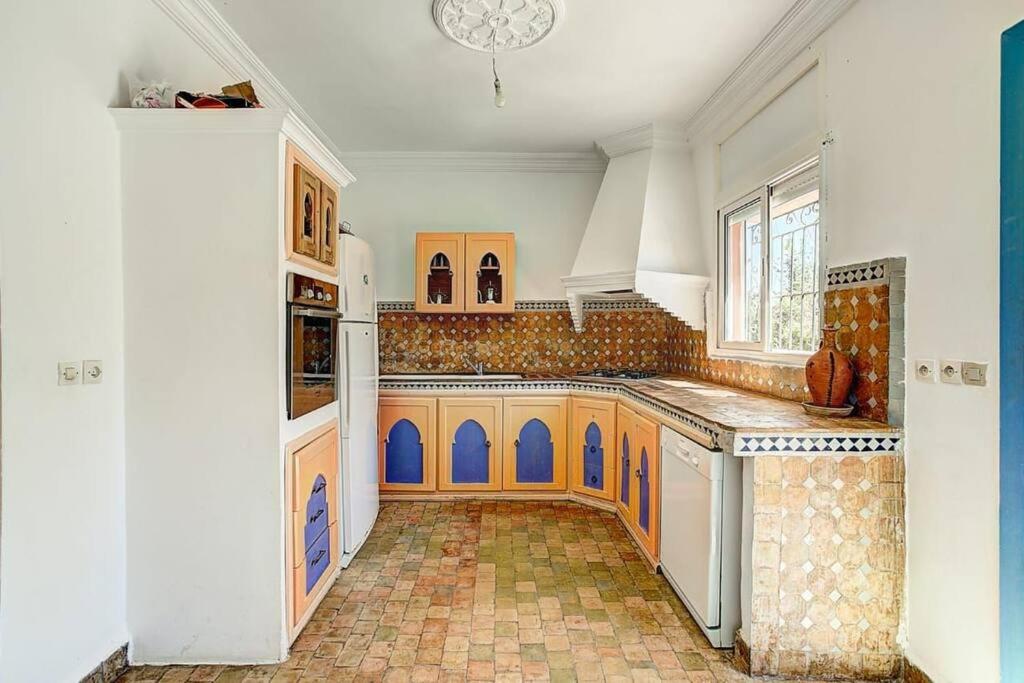This is a detailed photograph of a bright indoor kitchen featuring a unique blend of colors and textures. The kitchen floor is made of yellow and green bricks, providing an unconventional yet vibrant look. The walls are mostly white, creating a clean and airy atmosphere. A focal point of the kitchen is the lower cabinet doors, which are painted orange with a distinctive bright blue arched cutout in the center, reflecting a Moroccan style design. Above the countertop, which is tiled in a rust yellowish brown Mexican-style pattern, there are additional smaller cabinets. A white range hood extends from the corner to the ceiling above the stove. The kitchen has a variety of appliances including a white washing machine on the right-hand side, a built-in oven integrated with the cabinetry, and a small white refrigerator to the left. Above the countertop, there is a large window that fills the space with natural light. An ornate white circle adorns the ceiling, from which a lone light bulb hangs, adding a touch of simplicity to the ornate design elements of the room.